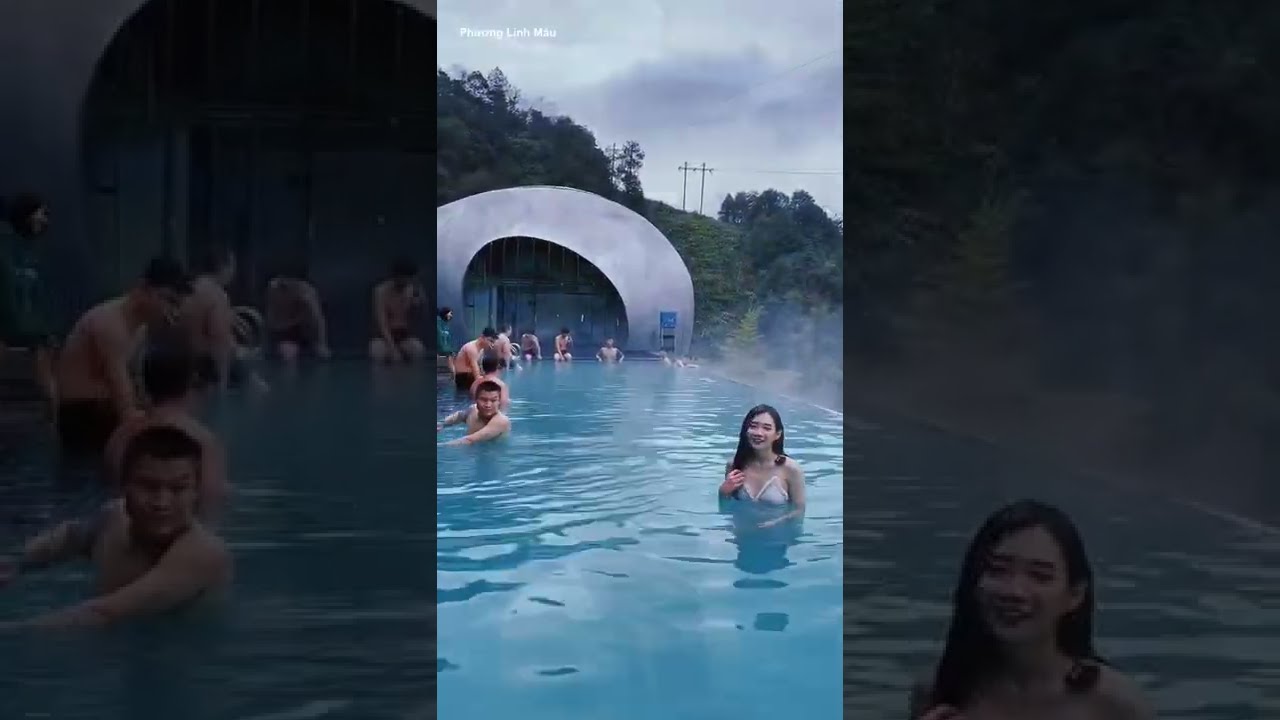This vertical outdoor photograph depicts a pool scene divided into three sections, with the central section in vibrant color while the sides are darker and muted. The pool, long and narrow, features vivid blue water emitting steam, likely due to a temperature difference with the cooler ambient air, indicative of a hot spring. At the far end of the pool stands a large gray dome-like structure with doors, beyond which lies a hillside with power lines cutting through a forest.

On the left and far end of the pool, several men, mainly shirtless and in trunks, are either sitting or leaning on the pool's edge. Prominently, a woman with long dark hair is positioned near the front right of the central section, smiling at the camera while partially submerged just below her white bikini top. Her dry hair suggests she hasn't been swimming. Her close-up appears on the right side of the image, reiterating her happy demeanor. In the left section, another man with dark hair, potentially directed towards her, adds further depth to the scene, while a possible watermark reading "Phuong Linh Mau" is visible in the top left corner. The combination of these elements paints a detailed and engaging depiction of a serene, steamy pool setting shared by relaxed individuals.